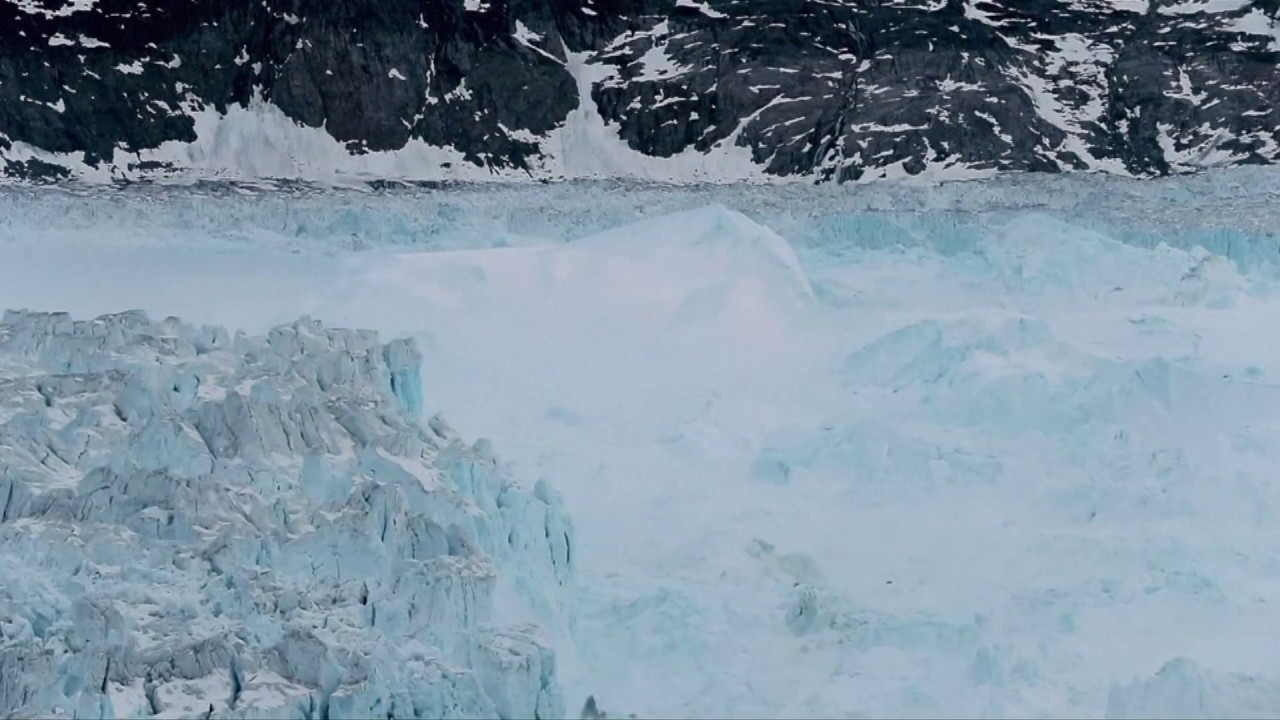The image captures a breathtaking landscape of a glacier set against the base of a formidable, almost sheer cliff of dark, craggy rock. The mountain in the background is dominated by nearly black rock, interspersed with patches of snow and ice, lending a textured, rugged appearance. The glacier itself occupies the majority of the frame with its striking, ragged expanse of bluish ice interspersed with white and gray chunks. A large, prominent white iceberg chunk forms a noticeable T-shape in the center, while the left side of the glacier reveals more detailed views of the individual rocks and ice chunks. The glacier’s surface varies in texture; the lower right side appears snowier, while the left is drier and more crusted. The overall color palette explores a mix of whites, light blues, and grays, illustrating the stark, raw beauty of this icy landscape.